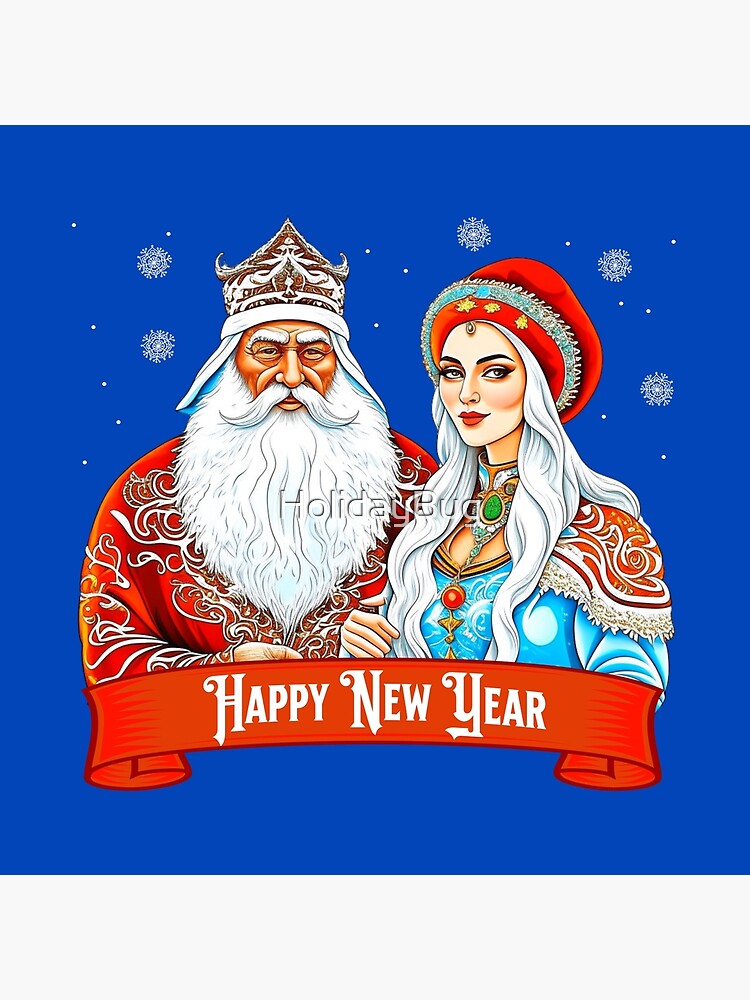The greeting card features a vibrant, cartoon-style illustration set against a bright blue background adorned with numerous white snowflakes and dots simulating snow. The foreground depicts two elaborately dressed figures resembling a festive rendition of a Russian Santa Claus and Mrs. Claus. Santa Claus, standing to the left, sports a big brown hat with white designs, a long white mustache and beard, and a tanned complexion. He is clad in a red coat with intricate silver trims, conveying a regal appearance. Beside him to the right stands Mrs. Claus, characterized by her youthful look, long white hair, and notable attire. She wears a red fluffy cap with gold and blue details and a matching red shawl over a blue dress. Her ensemble is accentuated by a large necklace featuring a prominent green and red stone. Both figures are positioned beneath a banner that reads "Happy New Year" in white letters, connected by a red ribbon. The watermark "Holiday Bug" is emblazoned across the main part of the image, which is depicted in high quality and free of any additional text.